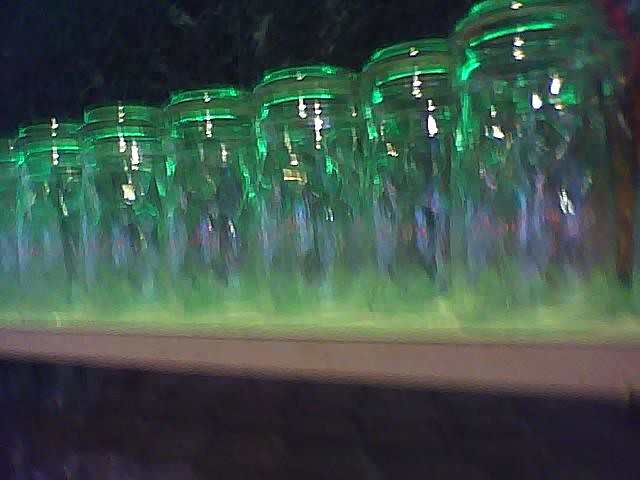The image appears to be a blurry photograph taken in a bar or restaurant, showcasing six empty drinking glasses lined up horizontally on a brown shelf. The glasses, placed upside down, have a greenish tint which seems to be influenced by the light source above them. The scene is set against a dark, almost black background, with a slight smoky effect in the top-left corner. The shelving unit holding the glasses is the only other visible element in the image. The glasses themselves have a glass lid appearance and are arranged in a single line, reflecting shades of green and yellow from the ambient lighting.